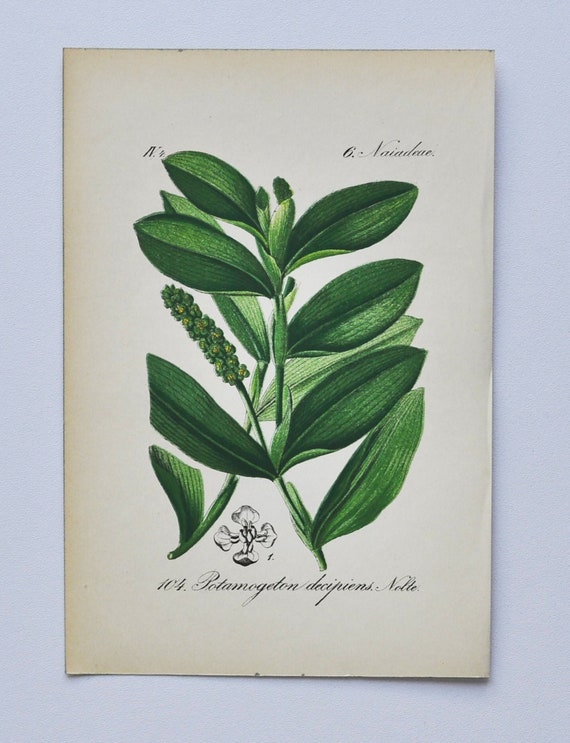This detailed botanical illustration, featured on a piece of weathered, light-brown-edged paper, depicts a large, verdant plant with cylindrical, dark green leaves. The paper, resting on a light blue surface, showcases the plant's intricate features, including stems with budding flowers that range from green to a lighter green hue. Against a gray background, the image also includes indistinguishable black cursive text in a Lucida-like calligraphy font, numbered as "104," with a partial etching of a floral petal at the bottom. A distinct small, cross-shaped symbol, adorned with floral ends and rendered in black ink, is visible on the page, further enhancing the ornate, vintage aesthetic of the illustration.